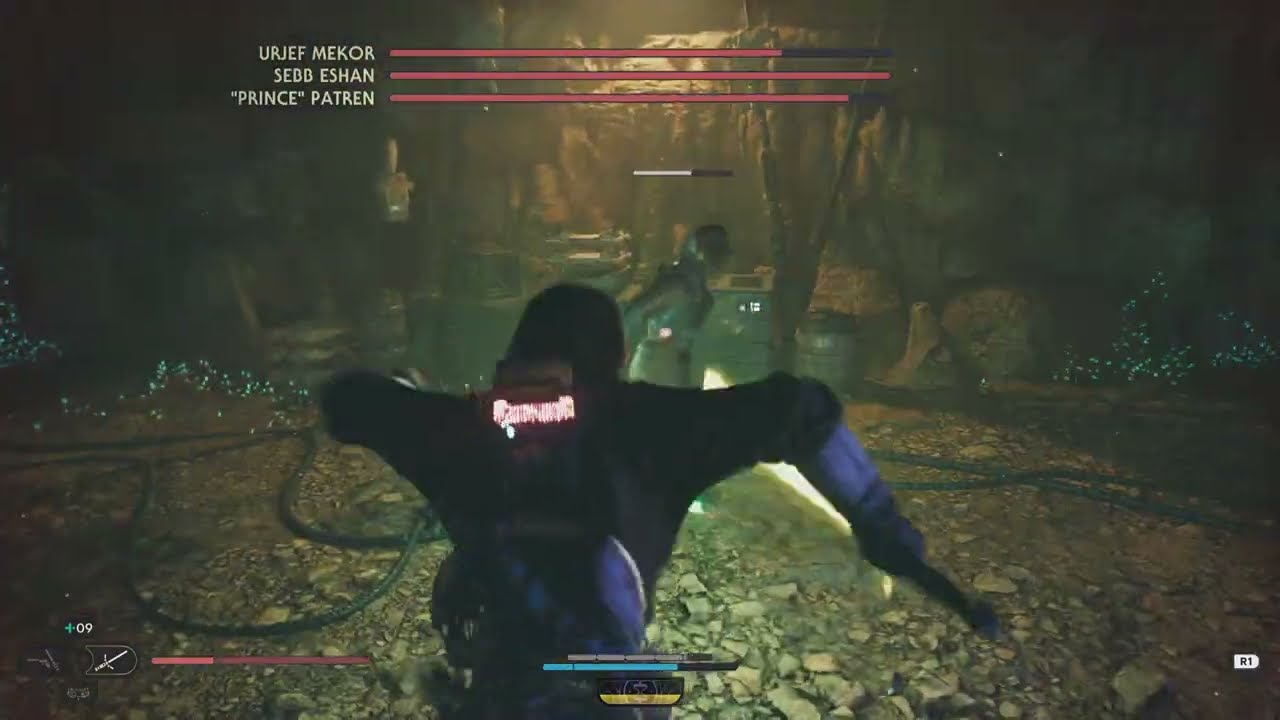This horizontal rectangular image is a slightly blurry screenshot from a video game set in a cave or stone building with predominantly brown and black tones. In the middle-lower portion of the image, the backside of an armored figure is visible. The armor is black and gray, and the figure is possibly human or creature-like, extending its arms outwards towards a blurry humanoid figure directly in front. This second figure appears to have brown and black gear.

The ground surface is rocky and dirt-filled, with some sporadic vegetation. Stone or rock walls form the background, contributing to the impression of a cave. At the top of the screen, three horizontal lines display white text: “you are Jeff Meekor,” “Seb Eshan,” and “Prince Patron” (with Prince in quotes). 

Additional game interface elements include a horizontal red bar with a small sword icon in the lower-left corner, representing health or resources, and a blue horizontal bar in the center of the screen. The lower right-hand corner features the text “R1.” The character in the image holds a neon green-yellow sword or lightsaber in his right hand and has a black backpack with indistinct neon pink writing. The setting and details suggest this is an action shooter game, with the character positioned centrally in the frame. The color palette includes black, white, red, tan, brown, green, purple, pink, and neon highlights, enhancing the immersive cave environment.